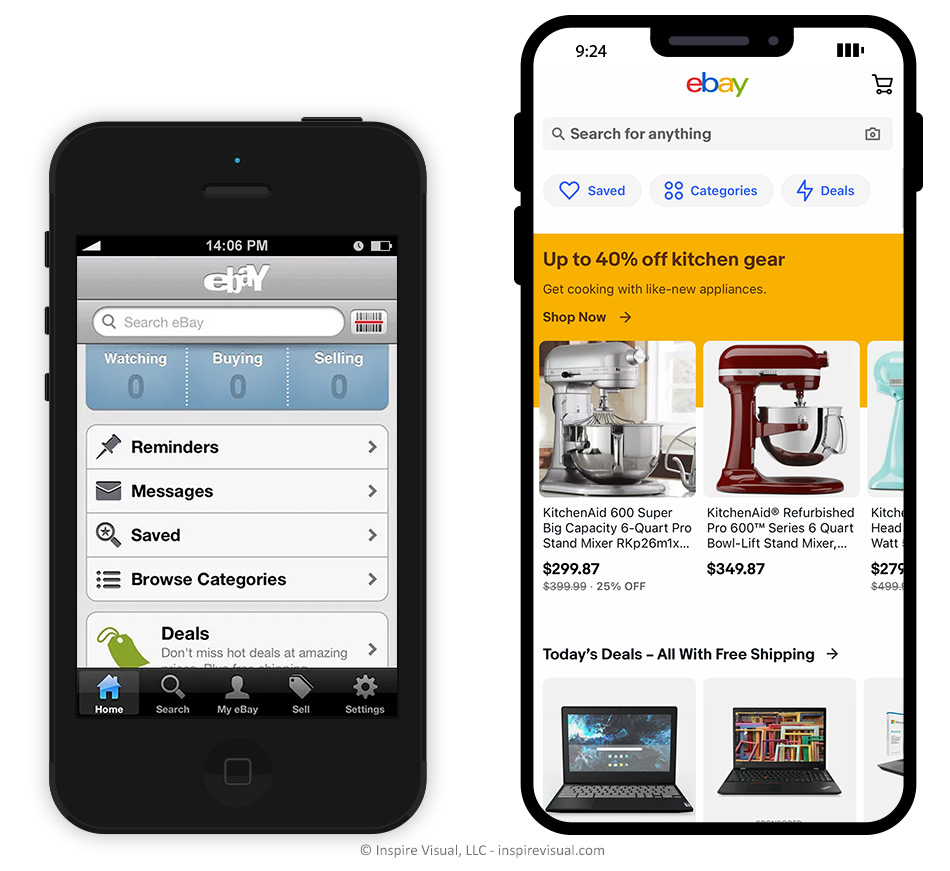The image features two mobile device screenshots showcasing a comparison between an older and a more modern version of the eBay mobile app. 

On the left side, the device is an older, smaller, black phone displaying an outdated version of the eBay site. The interface has a gray eBay logo at the top, followed by a search bar. Below that, there are three rectangular sections labeled "Watching," "Buying," and "Selling," each showing a count of zero. Further down, the interface includes expandable sections for "Reminders," "Messages," "Saved," "Browse Categories," and "Deals," as well as navigation buttons at the bottom of the phone screen. The entire layout appears antiquated and less user-friendly.

In contrast, the right side showcases a modern mobile device with a contemporary version of the eBay app. The redesigned interface features the colorful eBay logo at the top, alongside a search bar. Below that, there are clear shortcuts for popular categories such as "Saved Categories" and "Deals." The search results displayed include listings for mixers and laptops, indicating a more efficient and visually appealing user experience compared to the older version.